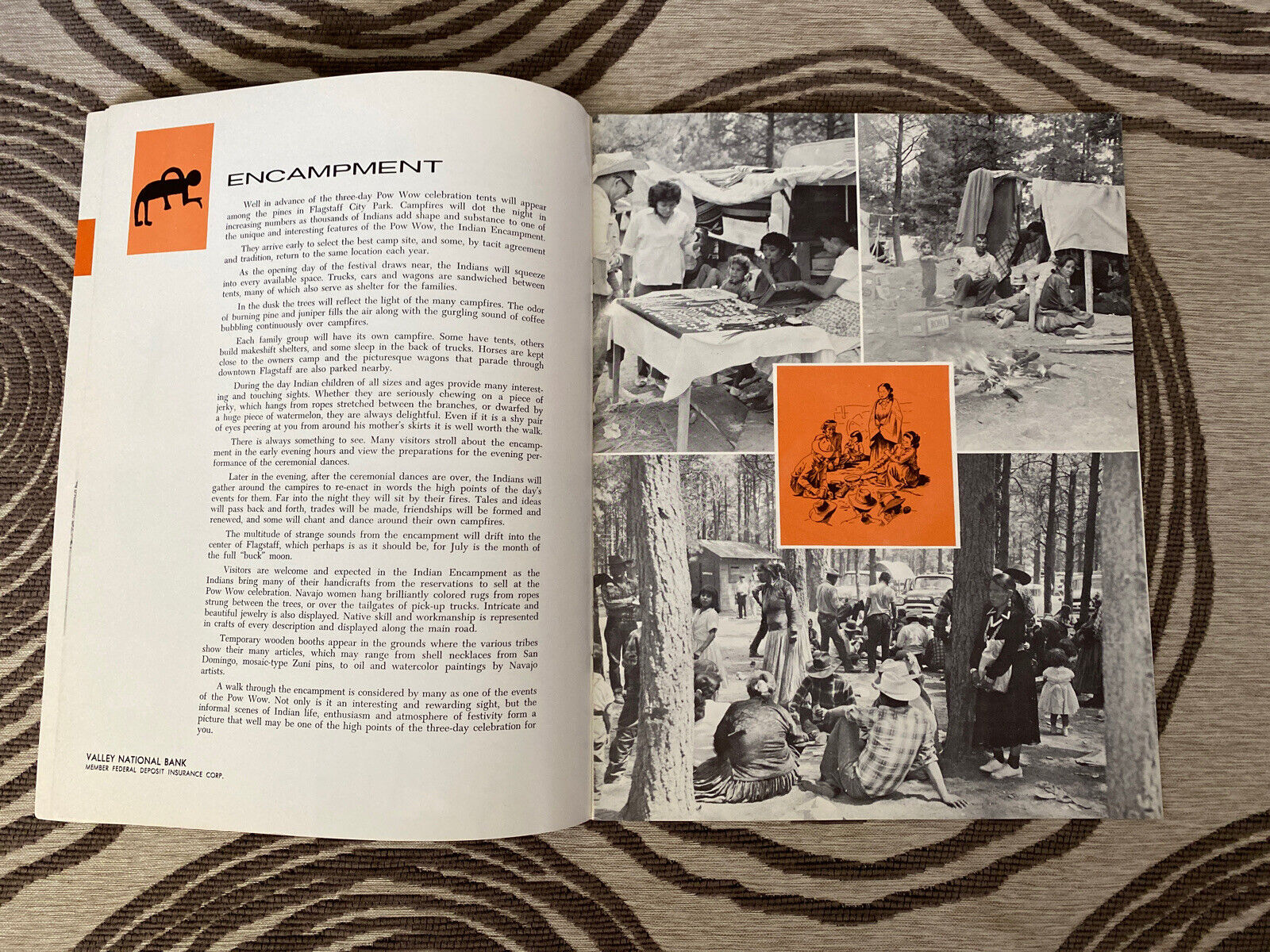An open booklet from the Valley National Bank, placed on a grey carpet with distinctive black ringed patterns, displays detailed imagery and text. The left page features an orange rectangle with a primitive drawing of a figure on all fours, beside the bold black title "Encampment," followed by an extensive text block. At the bottom left, the bank's name and an insurance mention are visible. The right page showcases three black-and-white photographs depicting an outdoor encampment scene, likely from the late 50s or early 60s. The top two images show groups of people around tables and an outdoor fireplace with makeshift tents made of blankets and sheets. The bottom photo captures a forest setting with flat ground, trees, and people sitting around, with cars visible in the background, suggesting a powwow celebration. Central to this page, an orange illustration with black drawings vividly portrays Native Americans in their encampment, accentuating the booklet's theme of traditional indigenous celebration.